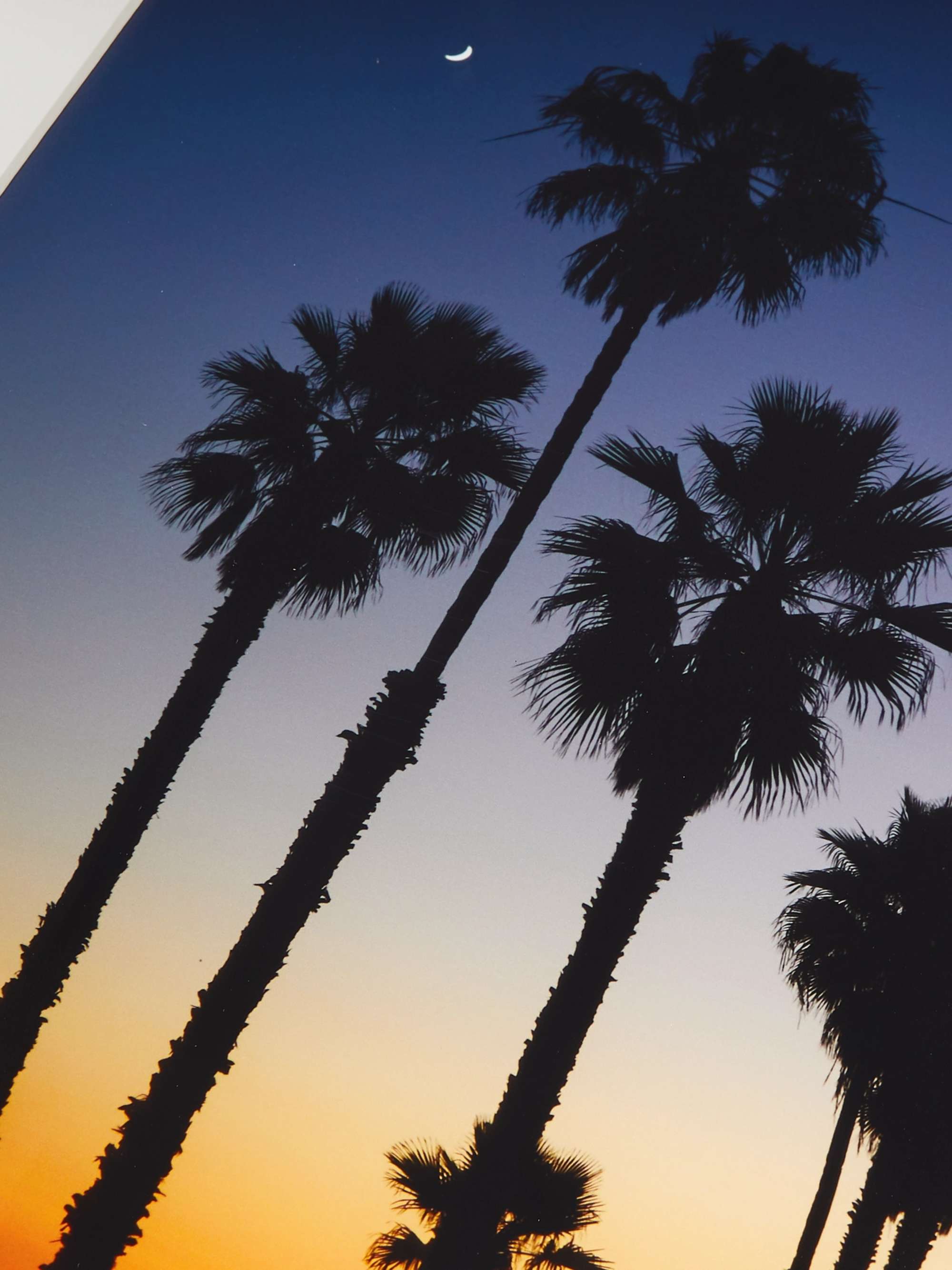This photograph captures a striking, tilted view of five palm trees silhouetted against a gradient sky at sunset. The image is taken from an unconventional perspective, where the camera is noticeably tilted, causing the trees to appear diagonal, stretching from the lower left to the upper right. The sky displays a beautiful transition of colors, with a deep, dark blue at the top evolving into a paler blue, then an amber glow, and finally a bright orange-yellow near the horizon. A small sliver of the moon is visible in the darkened sky. The upper left corner of the image is obstructed by what seems to be part of a ceiling or wall, suggesting the photo may have been taken just outside a house. The silhouetted palm trees stand tall with abundant palm fronds, creating a captivating contrast against the colorful backdrop.